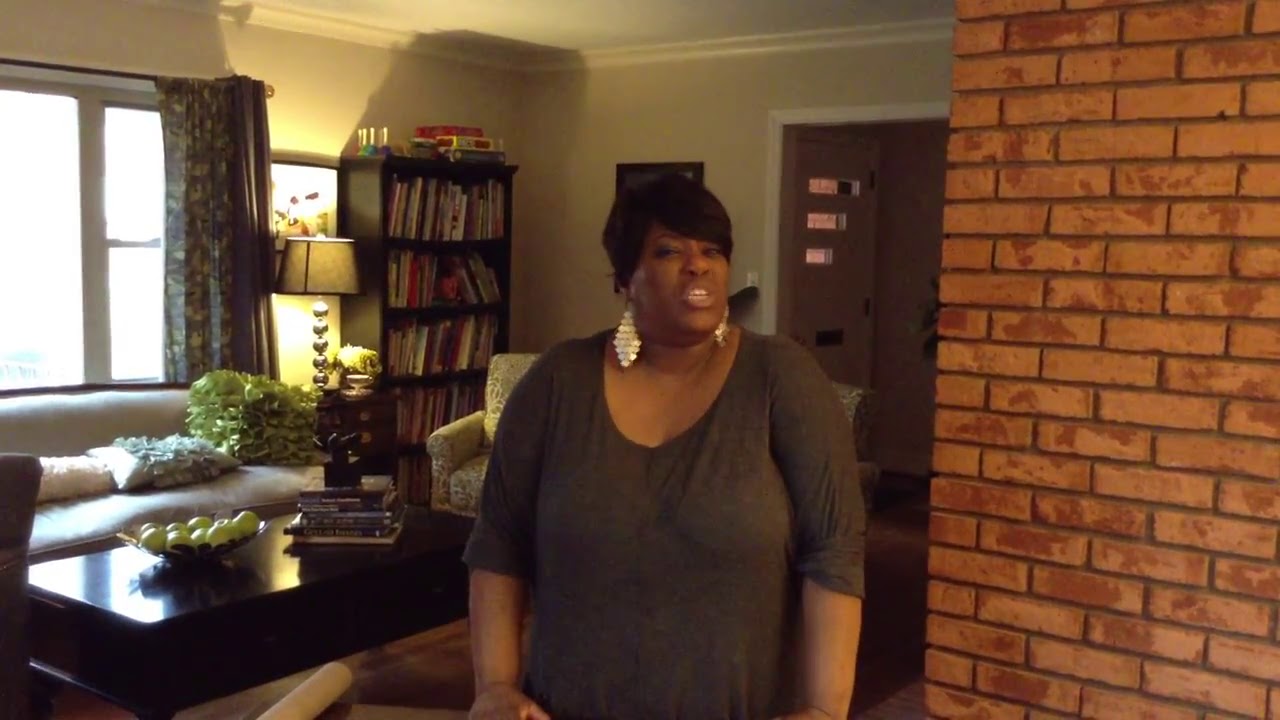The image displays a young black woman with short black hair in her living room, seemingly in the midst of recording a video for social media. She wears silver earrings and a gray shirt with the sleeves rolled up to her elbows. Her expression conveys distaste or disapproval as she squints toward the camera, her mouth slightly open as if about to speak. 

The well-lit living room features a mix of furniture and decor: a sofa, an armchair, a brick wall suggesting a nearby fireplace, and a marble table. The table holds a bowl of green apples or pears, a few other books, and additional items. A lamp, curtains, and a window with daylight streaming through are also visible. A bookshelf stacked with books is set against the wall, and a door can be seen in the background.